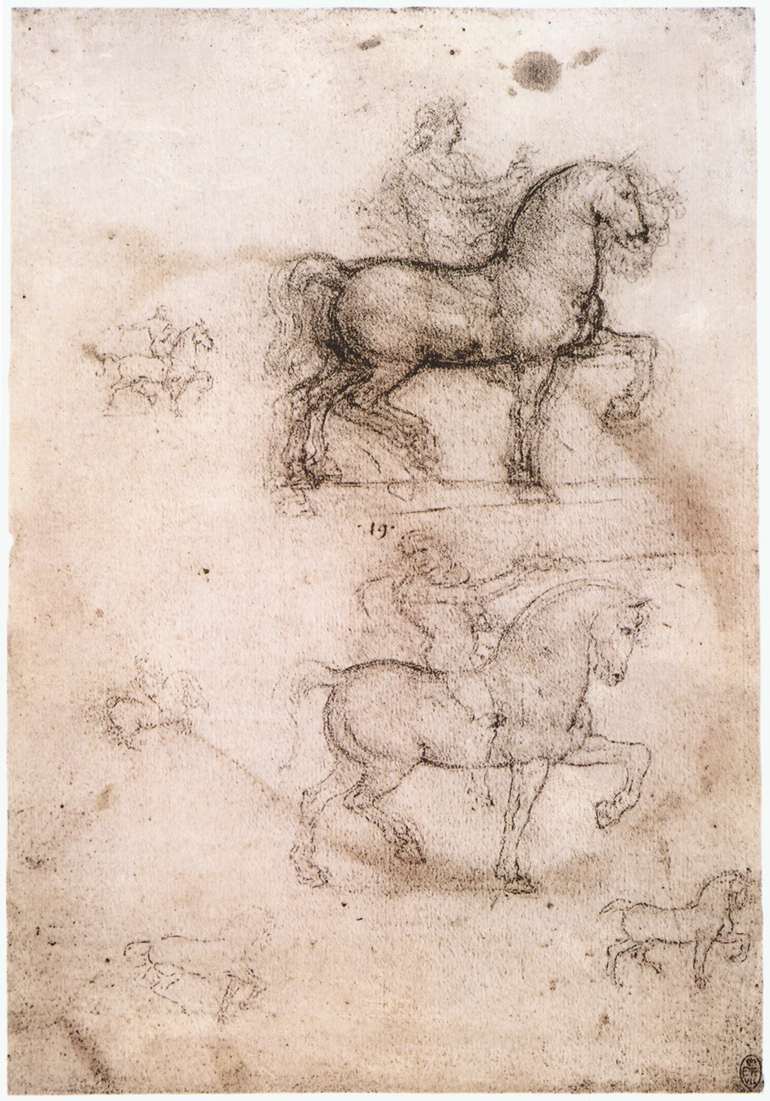This illustration comprises multiple sketches of horses and riders, drawn on aged, stained paper reminiscent of old-time treasure maps. Predominantly rendered in pen or charcoal pencil, the paper's wear adds a timeless quality to the composition. Central to the image are two larger, detailed sketches: the uppermost depicts a horse with shadows indicating different leg positions, and a rider wielding a sword, their left hoof raised and knee bent, suggesting movement. Directly beneath it, another horse and rider sketch exudes more refinement, with the rider appearing to point a gun. Around these, smaller, fainter sketches populate the page. On the left, vertically aligned images depict the horse running with a rider. Below the main sketches, two simpler drawings show horses in motion. Additionally, a label marked “19” appears above the second prominent horse, its significance unclear. The dynamic poses and varied completion levels of the sketches convey an artist's exploration of equine form and movement.